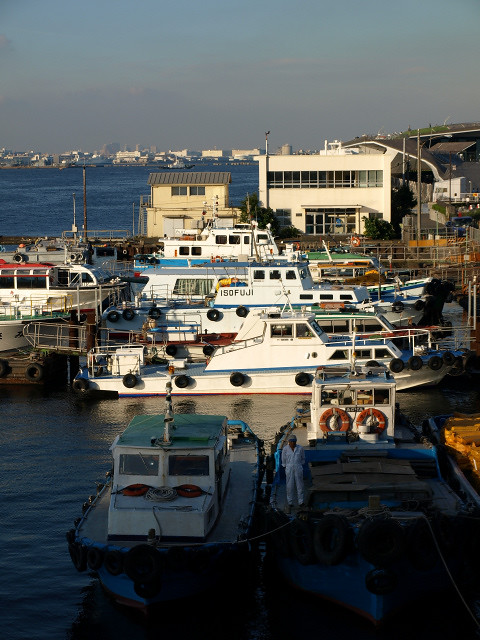The photograph captures a bustling marina or harbor scene, with a vast expanse of slightly rippling dark blue water in the foreground. The scene is framed by a slightly overcast, grayish-blue sky. The harbor is filled with various types of boats and yachts, tightly packed together, creating an almost busy visual tapestry. In the front center of the image, two prominently featured boats face opposite directions; the one on the right sports two life preservers with orange inner circles. Both have cabins suggesting they are passenger or small yacht vessels. A man in white coveralls with a baseball cap stands on the rightmost boat, adding a human element to the scene.

Aligned closely together, a mix of boats spans the middle of the image. Many of these are white yachts with front cabins and open backs, anchored at the docks. One visible boat bears the name "ISO FUJI." In the deeper background, a larger, older wooden fishing boat with a cabin stands out along with a houseboat. 

Nestled in the background are several buildings— a two-story beige structure with a gray roof and a taller white building resembling an office space with glass doors and windows. These buildings are flanked by docks, indicating a commercial or industrious setting, potentially where dockmasters operate. Farther back, the skyline of a city along the shore can be discerned, cementing the blend of industrial and maritime life. Off to the right, there appears to be what looks like a bridge or elevated roadway. Overall, the photo richly details a vibrant, activity-filled marina against the backdrop of an overcast urban skyline.